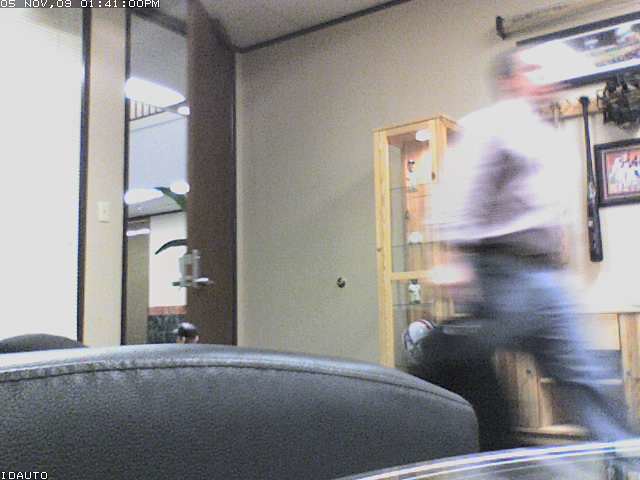A man with short black hair, wearing a white button-down shirt and blue pants, is captured in mid-stride as he exits an office, a black backpack slung over his shoulder. The motion in the image is evident from the blur across his legs and body. He appears to be a Caucasian male and is walking past a display area within the office. To his right, there’s a showcase featuring a black baseball bat, a catcher's mask, and a framed picture, though the details of the picture are indistinct. Adjacent to the display, there's a glass case containing various memorabilia. The background also includes a large leather love seat or couch and a gray chair. An open door reveals a glimpse of another section of the office, illuminated and housing a green plant.